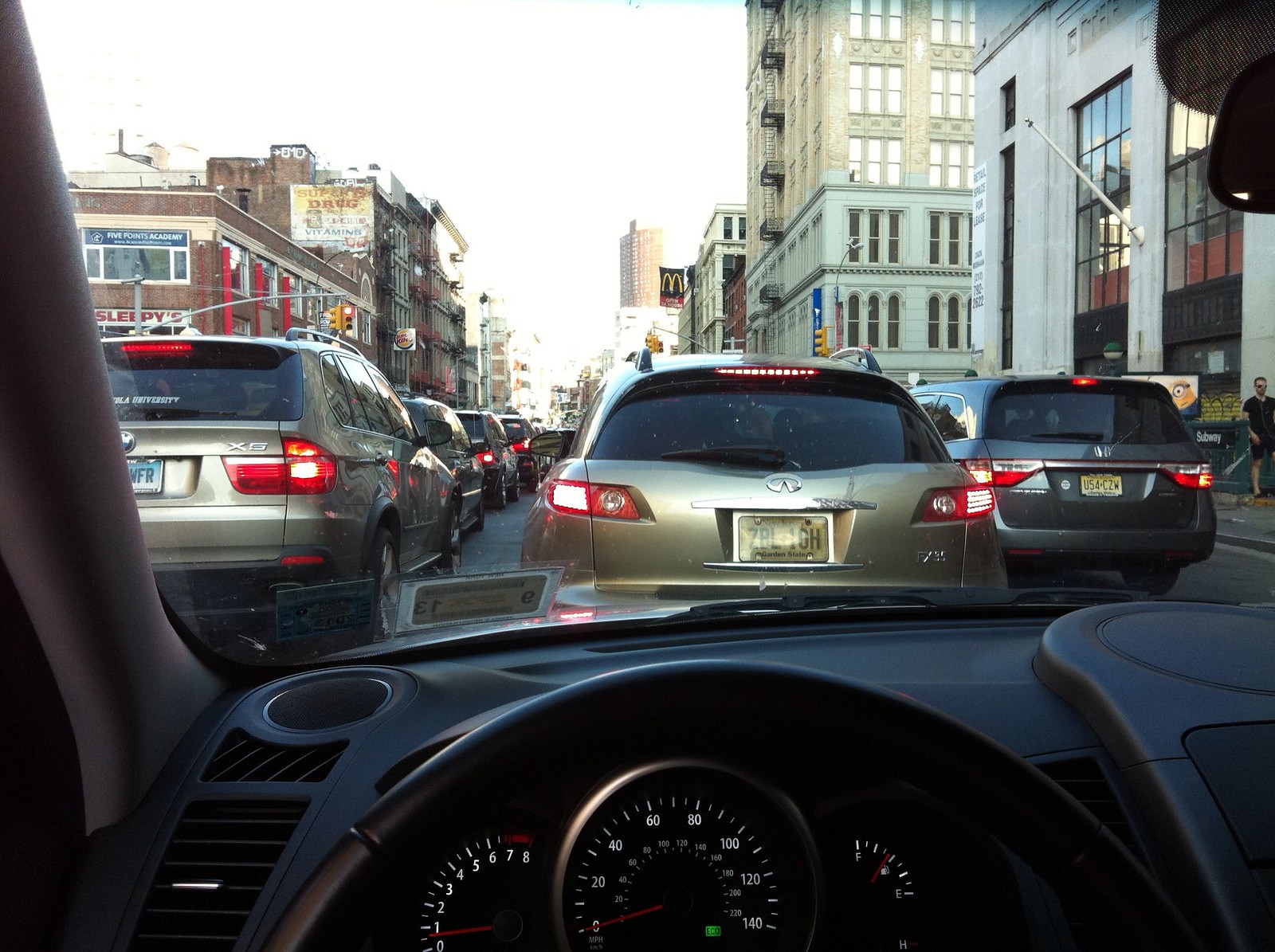The image captures a scene from the driver's seat inside a small vehicle, showcasing a downtown urban area during a sunny day. You can see the black steering wheel and a detailed dashboard with illuminated white numbers on the speedometer that ranges from 0 to 140, the RPM tachometer running from 0 to 8, and the fuel gauge. The car's interior feels compact but modern. 

Through the windshield, there's heavy bumper-to-bumper traffic spanning three lanes. Directly ahead, multiple vehicles are visible, including two gold-colored cars and a grayish van. The traffic is dense and extends as far as the eye can see. Prominent signs in the scene include a McDonald's logo in the center of the picture, a Burger King sign, and a somewhat faded Superdrug sign with the word ‘vitamins’ beneath it. There's also a Sleepies sign on the left-hand side, and a banner for Five Points Academy is noticeable in one of the building windows. 

The urban backdrop features several tall buildings with numerous windows. On the right, there's a residential building equipped with fire escapes, and a bank-like structure with a flagpole. A sidewalk runs along the side where a pedestrian can be seen walking. Overall, the scene is lively yet static as all vehicles are at a standstill, likely waiting at a red light.